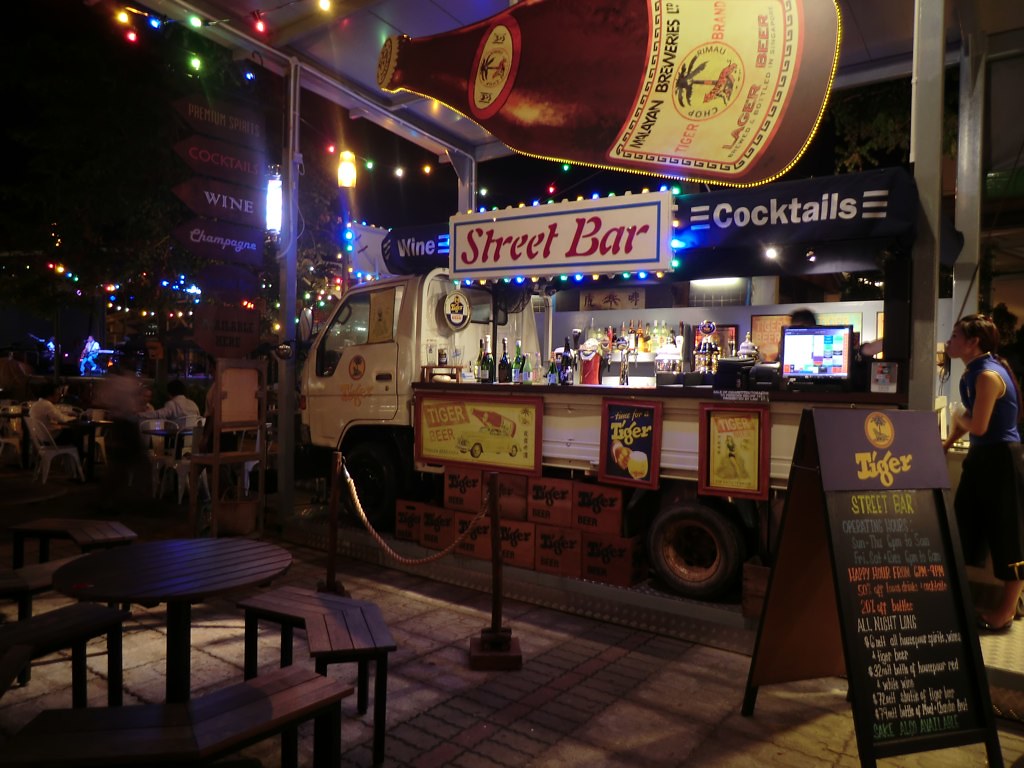This is a nighttime color photograph taken outdoors in a city, capturing a vibrant street scene centered around a unique cocktail truck called "Street Bar Cocktails." The truck, standing at an angle, has been converted into a fully equipped bar. It features an extensive setup with signs advertising drinks such as "Tiger Street Bar," "All Night Long," and "Happy Hour." Above the truck, there's a large cutout of a beer bottle labeled "Malayan Breweries, Lager Beer," depicting a palm tree. Adding to the festive atmosphere, a tall 15-foot sign in the background reads "Champagne, Wine, and Cocktails."

Surrounding the truck, numerous colored string lights of brown, red, yellow, blue, green, orange, and white create a warm and inviting ambiance. There are tables and chairs scattered around, with several patrons visible in the distance enjoying their drinks. To the truck's side, some lights are either ceiling-mounted or attached to umbrellas. One of the tables at the bottom left is empty, while a customer can be seen at the back right of the bar. The scene is lively, detailed with various menus and round tables, making it clear this is a popular spot for an evening out. In the background, more people can be observed seated at tables, adding to the bustling nightlife atmosphere depicted in the photograph.